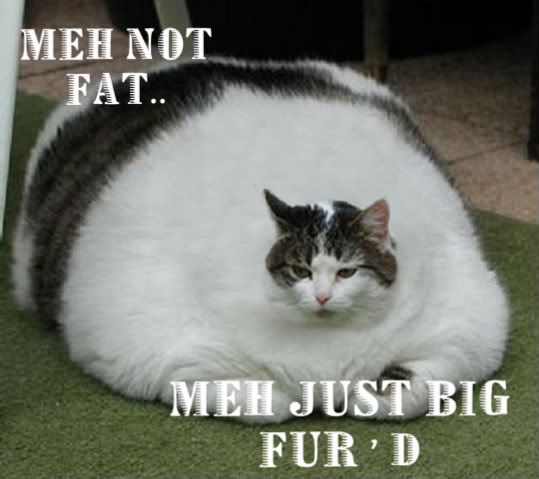The image is a satirical internet meme watermarked by Photobucket. It features an excessively large cat, appearing 15 to 20 times bigger than a typical cat, with its head disproportionately small relative to its massive body. The cat is gray, black, and white with a head comprising these colors in a mixed pattern. Surrounding the head, the body shows alternating bands of white and gray-black fur, giving the impression of an enormous girth. The text in the meme reads at the top in capital letters, "MEH NOT FAT," and at the bottom, "MEH JUST BIG FURRED," humorously suggesting that the cat's size is due to its fur. In the middle of the image, a white bar carries the phrase, "PROTECT MORE OF YOUR MEMORIES FOR LESS," as part of Photobucket’s watermark. The cat is lying on astroturf, looking slightly perplexed, with green eyes and ears perked up. Behind the cat, there is a tiled floor and what appears to be a bench or a piano. This meme effectively combines humor and exaggerated imagery to entertain viewers.